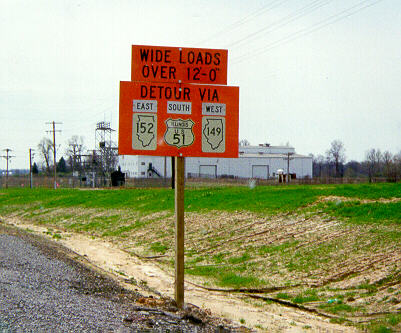This color photograph captures a roadside detour sign prominently displayed on a tin metal pole. The sign is predominantly red with sections of white containing various symbols and numbers at the bottom. The main text on the red background reads, "Wide Load Over 1201 Detour." Below this, there are three symbols, possibly depicting maps and numbers or other symbols.

To the left of the sign, a dark blue road stretches into the distance. The immediate background behind the sign features a strip of green grass verge, transitioning into a sandy and barren area towards the edge. Further back, a white building stands centrally behind the sign. Power lines extend from the left side of the image and span across the sky. The sky is predominantly clear with a greyish hue, showing hints of blue at the top right corner. Additionally, the far right edge of the image includes some trees, adding a touch of natural greenery to the scene.